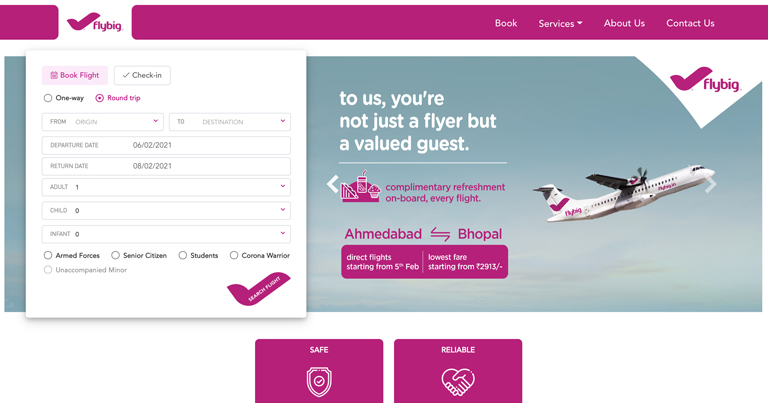Screenshot of the FlyBig website

The FlyBig website displays a vibrant magenta theme with a distinct purple header. On the left side of the header, there's a white field featuring the FlyBig logo, which is presented in lowercase letters. Adjacent to this, there's an airplane icon that cleverly doubles as a check mark, with the fuselage pointing upwards and the tail angled to the side. 

To the right of the header, a menu provides options for "Book," "Services" (which includes a drop-down menu), "About Us," and "Contact." Below the header, two purple buttons, labeled "Safe" and "Reliable," are adorned with icons of a shield and two hands shaking, respectively.

The hero section prominently displays an image of a mid-sized propeller airplane, commonly referred to as a commuter or puddle jumper plane. The aircraft is angled upward at about 15 degrees against a backdrop of clear sky, positioned on the far right side of the image. 

Beneath the hero image, there is a white drop-down area with options for booking flights and checking in. The booking options include "One Way" and "Round Trip," with "Round Trip" being selected in a darker purple hue. Users can enter their departure and return dates as well as specify the number of adults and children traveling. Additional checkboxes allow for special categories such as armed forces personnel, senior citizens, students, and corona warriors.

To the left of the airplane image, text emphasizes the airline's customer commitment with the message, "To us, you're not just a flyer but a valued guest." Icons representing complimentary refreshments highlight the onboard perks offered by FlyBig. Further down, a promotional offer details direct flights from Ahmedabad to Bhopal starting on February 5th, with the lowest fare listed at ₹2,913.

Overall, the website combines a visually appealing design with user-friendly navigation, aimed at providing a seamless and informative booking experience.